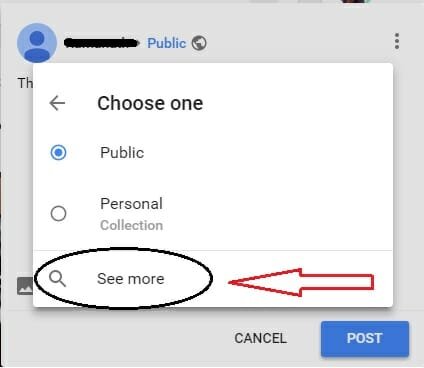This image is a square screenshot of a digital interface—possibly from a blog or social media platform. The central focus of the screenshot is a user post interface. At the top left, there is a circular icon representing a user, though the name associated with this icon is crossed out. Next to the icon, there is a label that says "Public," accompanied by a globe icon, indicating the post's visibility settings. To the right of the public label, there is a three-dot vertical menu icon.

Below this header section, there is a text box for the post content. At the bottom of the text box, two buttons are visible: a grey "Cancel" button on the left and a blue "Post" button on the right. Overlaying this interface is a white pop-up window with a drop shadow, adding a layered effect. The pop-up window features a back arrow on the top left and the text "Choose one" followed by two options: "Public" and "Personal." The "Public" option is selected, indicated by a blue beacon icon, while the "Personal" option, labeled as "Collection," is unselected and displayed in grey text. Below these options, there is a search bar with a magnifying glass icon, followed by the text "See more," all under a thin grey line.

The pop-up window and the underlying post area have been highlighted with a very pixelated black oval, and a heavily pixelated red arrow points to this oval from the right, presumably to draw attention to it. The background of the underlying post area is light grey. A tiny, barely noticeable section of an image, possibly a JPEG, peeks in from the top and left edges of the screenshot, but it is too small (only a few pixels on each side) to identify.

Overall, the image illustrates a layered user interface with a focus on choosing the visibility settings for a post, enhanced by rudimentary annotations that crudely emphasize certain interface elements.